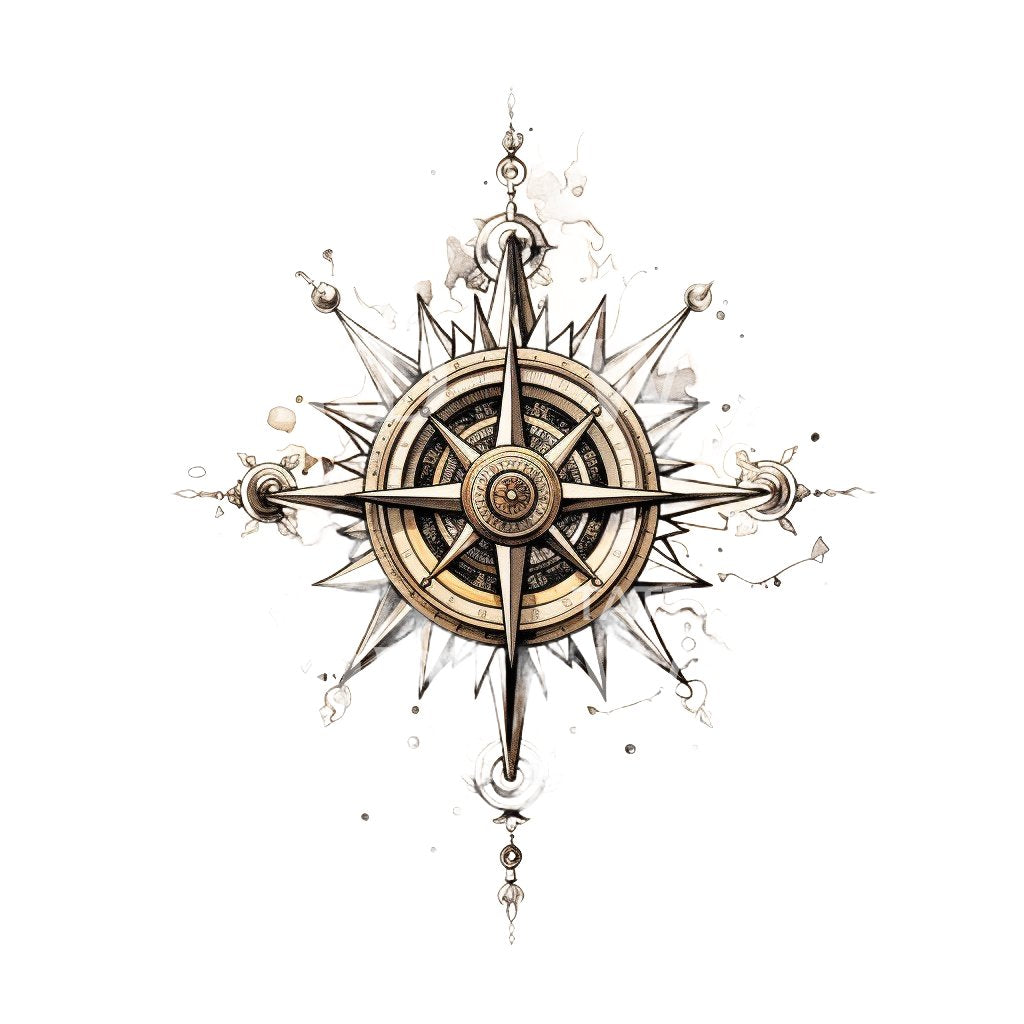The image is an intricate, computer-generated artistic design of a compass set against a solid white background. Dominating the center is a sequence of concentric circles: a prominent gold outer circle, a lighter gold circle inside it, followed by a darker gold circle, a textured black circle, another solid gold circle, and finally, a smaller gold circle at the heart of the design. Radiating from the central circles are gold arrows pointing in the four cardinal directions (north, south, east, and west) and four ordinal directions (northeast, northwest, southeast, southwest), forming a star-like pattern. Surrounding these central points are additional outlined spikes varying in length, shaded in white and gray with black outlines, extending towards the outer edges and further accentuating the compass's detailed and symmetrical design.